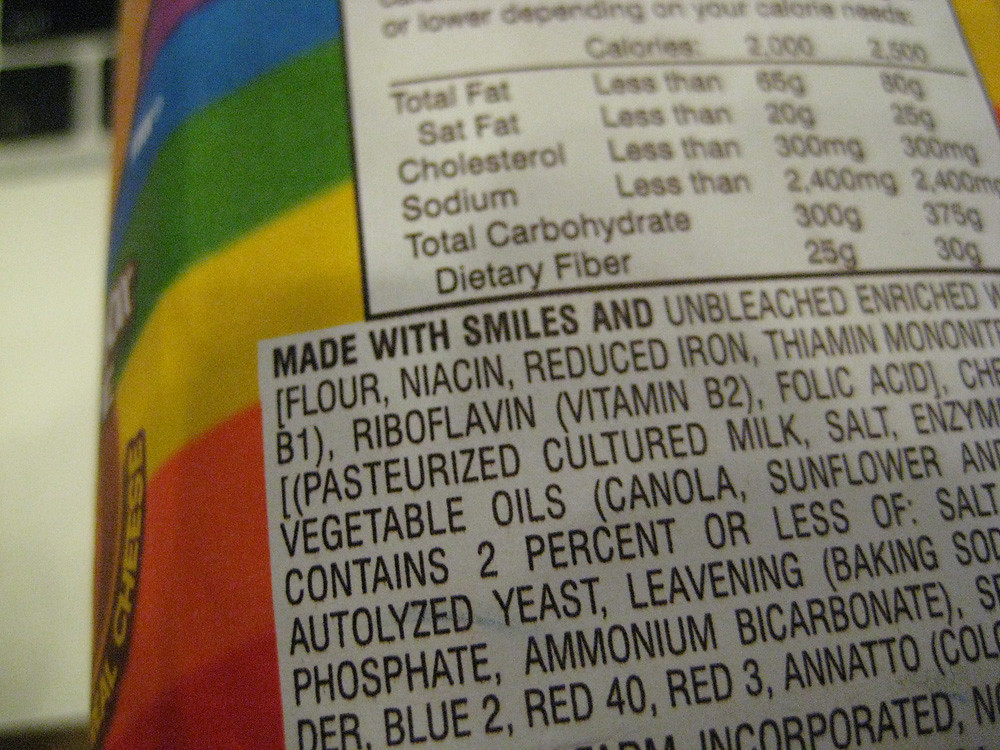Close-up photograph of a bottle with a black background. The bottle features vibrant, rainbow-colored stripes in purple, blue, green, yellow, orange, and red. Initially appearing to be a drink or vitamin beverage, the label reveals it to be a cheese product with "Real Cheese" prominently displayed. The label also lists ingredients, including unbleached enriched flour and various chemicals, alongside the phrase "Made with smiles."